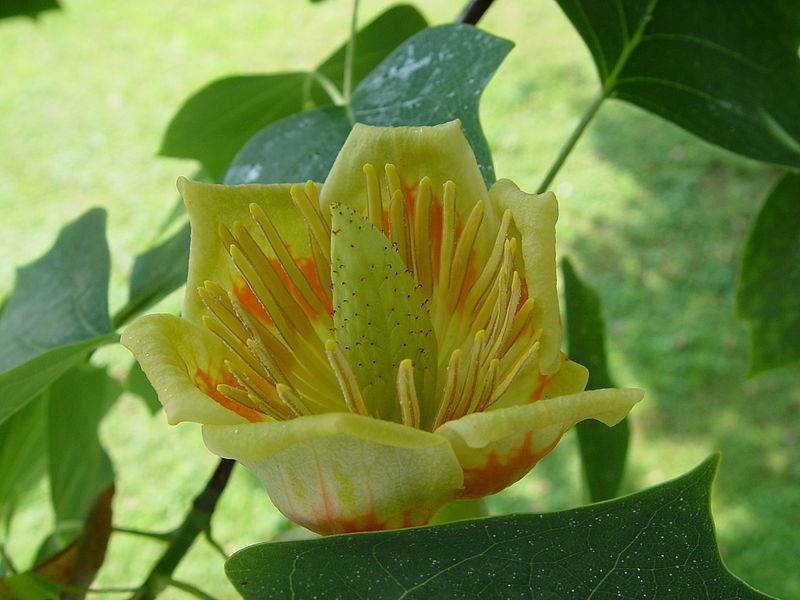This rectangular outdoor photograph, taken on a bright sunny day, captures the vibrant essence of nature. The focal point of the image is a stunning, nearly-blooming yellow flower with petals that are pale yellow, curling delicately at the tips, and tinged with shades of peachy orange at their base. Six main petals radiate outwards, surrounding a central structure with a complex array of features. At the core of the flower is a long, tongue-shaped area, pale yellow with a hint of green, adorned with tiny red and brown specks. From the base of this central structure, numerous slender, straight yellow filaments extend outwards, possibly serving a pollination function. This intricate flower is surrounded by large, dark green, pointed leaves that provide a lush backdrop. The background further highlights the natural setting, featuring a soft, light green grassy ground that adds to the overall serenity of the scene.